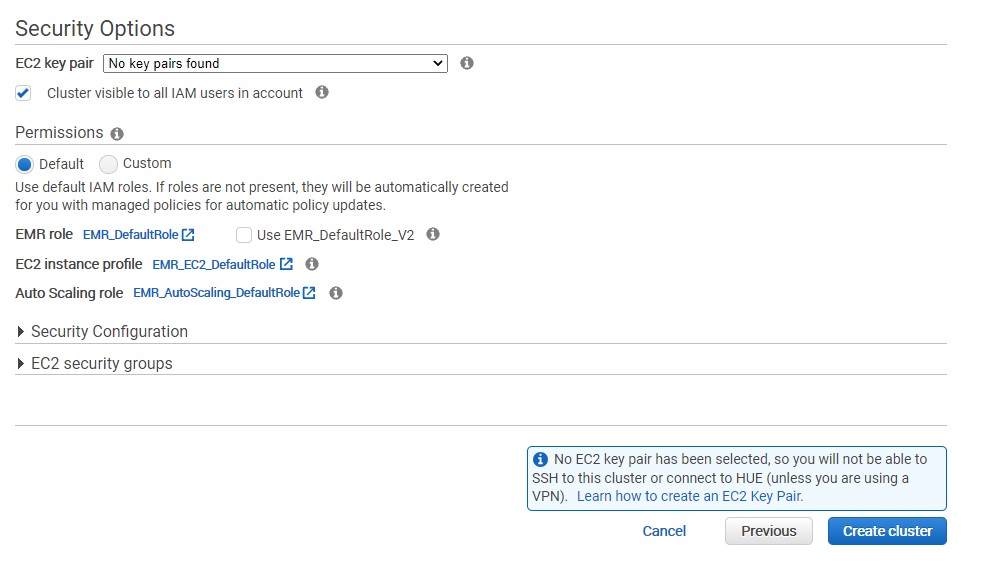Here's a detailed and cleaned-up descriptive caption for the image:

---

**Security Options Overview**

The screen displays the "Security Options" settings for an unidentified device. The first section is titled "EC2 Key Pairs" and states, "No key pairs found." This section includes a dropdown icon and a round, dark circle with a small 'i' inside, indicating additional information is available.

Below this, there's a checkbox marked "Cluster visible to all IAM users in account," accompanied by the same information icon.

The next section, labeled "Permissions," includes an information icon. Within this, the "Default" option is selected, denoted by a dark blue highlight, while the "Custom" option remains unselected, shown in white. The text clarifies: "Use default IAM roles. If roles are not present, they will be automatically created for you with managed policies for automatic policy updates." The roles listed are:
- **EMR Role**: `EMR_default_role` (in blue, indicating a link)
- **EC2 Instance Profile**: `EMR_EC2_default_role` (also in blue)
- **Auto Scaling Role**: `EMR_auto_scaling_default_role` (in blue)

Additional clickable options are available through forward arrows for "Security Configuration" and "EC2 Security Groups."

At the bottom right of the screen, a blue rectangular box with an information symbol states: "No EC2 key pair has been selected, so you will not be able to SSH to this cluster or connect to HUE unless you are using a VPN. Learn how to create an EC2 key pair" (the latter part is in blue and likely clickable).

Finally, navigation options include "Cancel," "Previous," or "Create Cluster."

---

This caption provides a clear and structured description of the image, detailing all visible elements and their functions.